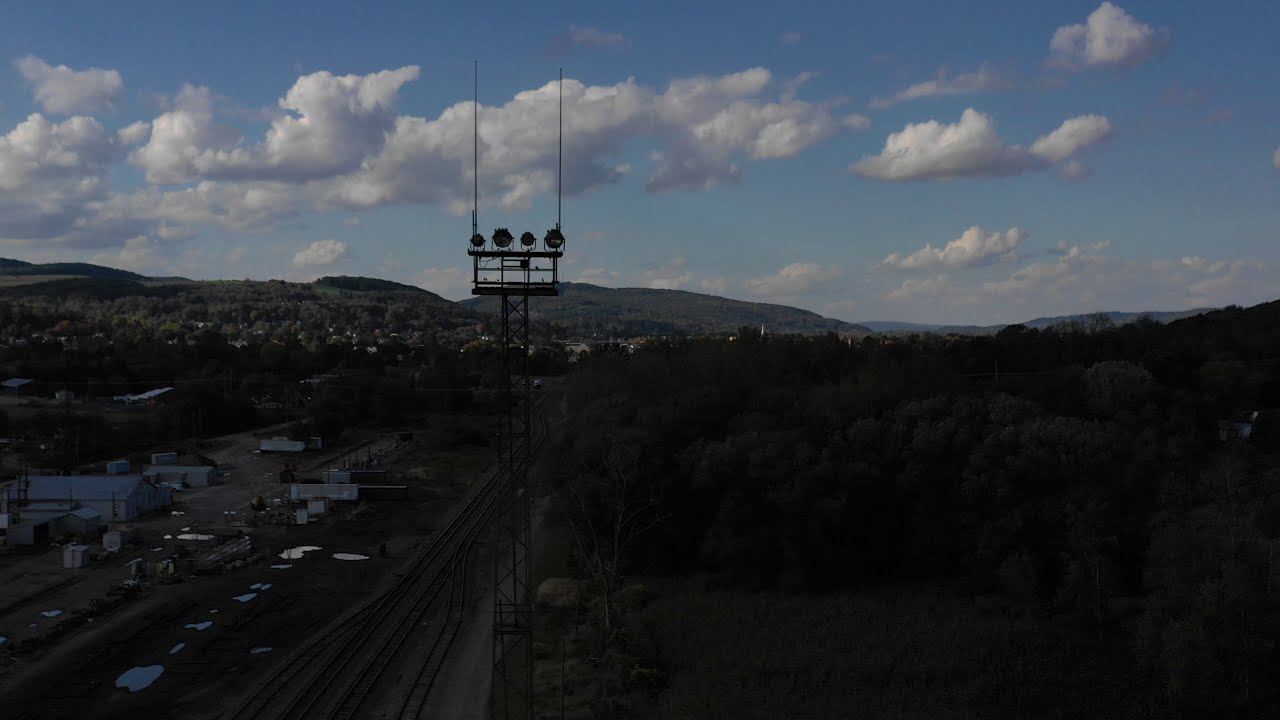This drone-captured image, taken from an elevated position outdoors, presents a striking landscape scene under an overcast sky. The darkened ground, shrouded in shadow due to the dense cloud cover above, sharply contrasts with the bright blue sky and its decorative white and gray puffy clouds. Dominating the center of the image, slightly to the left, stands a tall antenna tower featuring four round black objects on its top and a few crossbars in the middle. Below, a set of train tracks bisects the scene, dividing the dense, dark green forest into two halves. To the left of the tracks, a few plain white outdoor buildings punctuate the shadowed land. In the background, rolling hills and mountainsides covered in trees extend into the horizon. The primary colors in the image are blue, white, brown, black, and shades of gray, which together create an evocative and moody atmosphere highlighting dramatic contrasts between light and shadow.